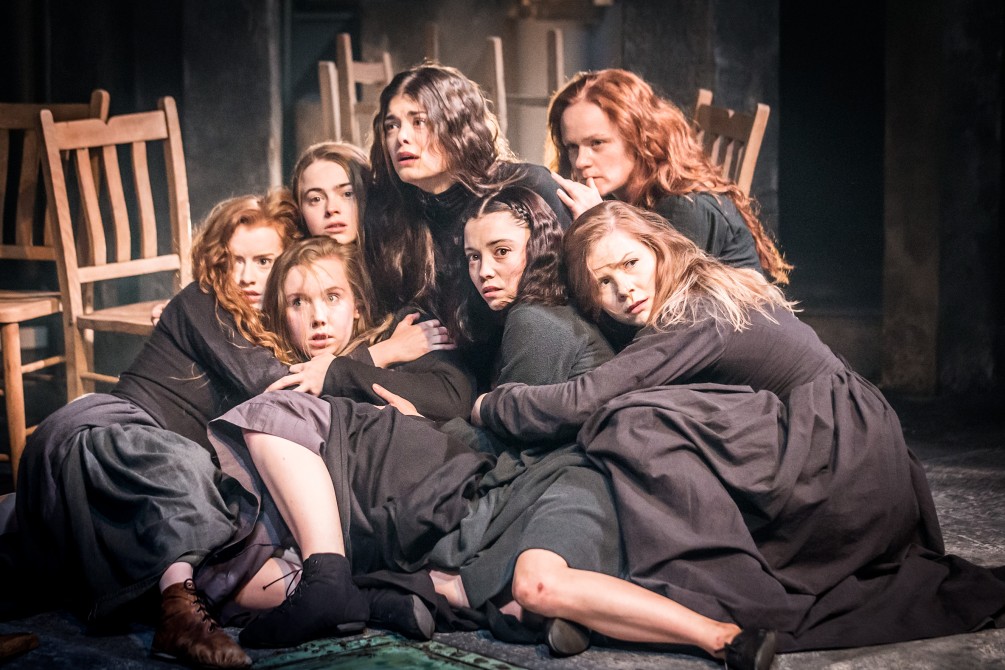In this rectangular photograph, we see seven young women, likely ranging from ages 13 to early 20s, huddled together on a dark stone floor. They are wearing identical long-sleeve black dresses with tight-fitting tops and loose, flowing skirts, evoking attire from a different historical period. The girls, all Caucasian, exhibit expressions of fear and anxiety, their faces showing clear terror as they cling to each other. Some are gazing upwards, while others look around with focused intensity. The scene behind them is cluttered with brown wooden chairs, some overturned, adding to the chaotic atmosphere. The upper right corner of the image is shadowed, contributing to the overall sense of foreboding.